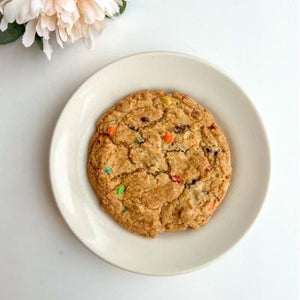In the image, a single large, circular chocolate chip cookie adorned with colorful specks of green, red, orange, blue, and brown sits on a small white plate. The specks might be M&M pieces or possibly dried fruit, adding bursts of color to the well-browned, cracked surface of the cookie. The plate rests on a white table that blends seamlessly into the white background. In the upper left-hand corner of the image, part of a flower, which appears to be a carnation, along with its green leaves and some white and peach blossoms, subtly intrudes into the frame, adding an elegant touch to the otherwise minimalistic setting.